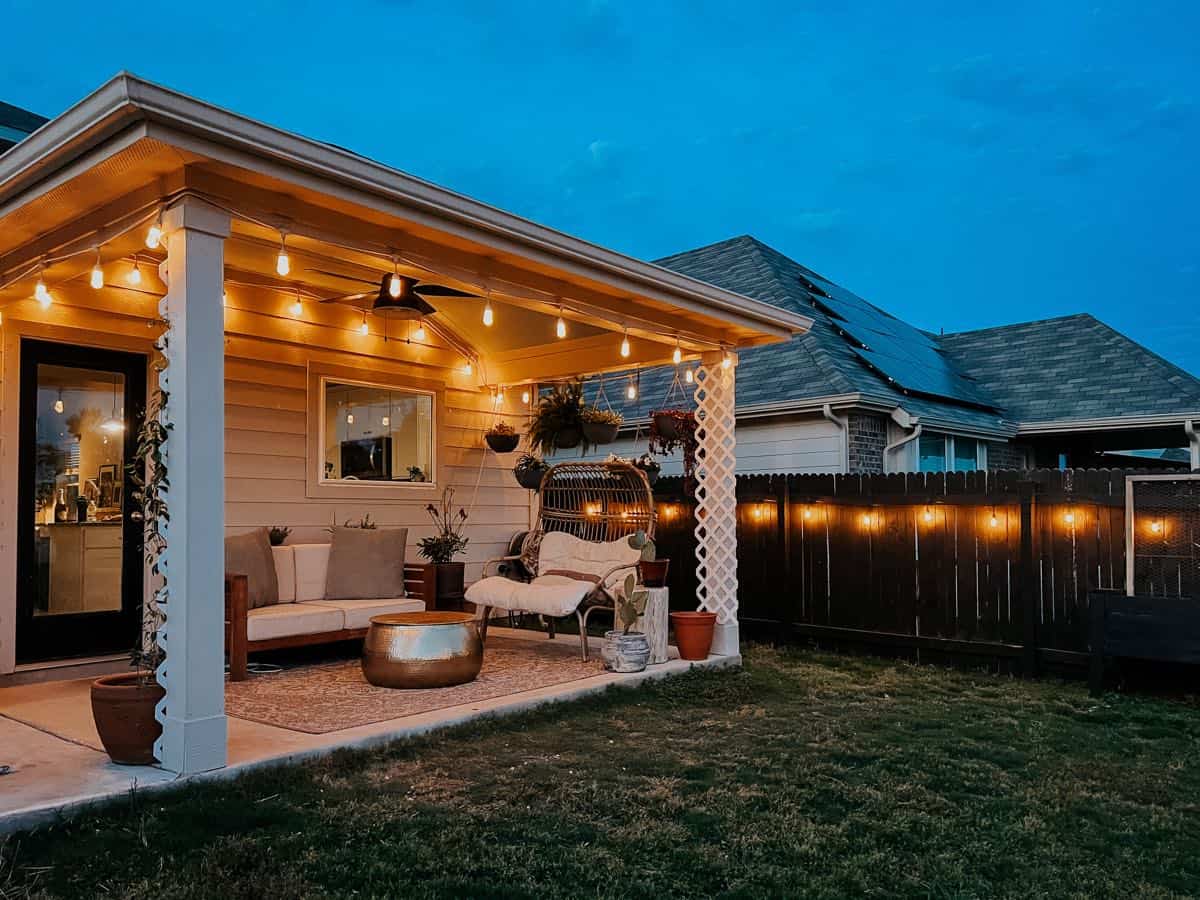An evening twilight captures the cozy ambiance of a front porch, nestled under an extended roofline with corner support pillars adorned with white diamond-shaped trellises. Large plant pots, one red and another white with a thriving green plant, rest at the base of these pillars. The broad concrete patio is elegantly decorated with a light tan, ornate rug beneath a stylish white outdoor sofa featuring large pillows and a wooden frame. Adjacent is an ornate patio table, possibly crafted from semi-cylindrical brass, and a cushioned wicker lounge. The house, a white wood frame structure with a screen door leading into the kitchen, is animated by numerous electric lights strung along the porch’s roof edge and the brown wooden privacy fence. An outdoor ceiling fan complements the ambiance, while the lawn, though slightly dried, adds a touch of natural charm. On the other side of the fence, a neighboring house with gray and black brick and rooftop solar panels completes the picturesque setting under a twilight sky with scattered blue clouds.